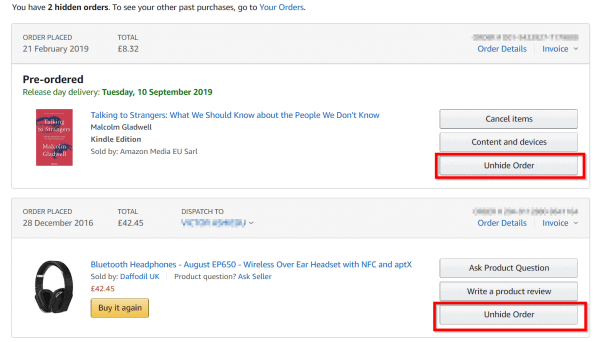Screenshot Description: Amazon.com Order History with Hidden Orders

The screenshot features a section from an Amazon.com order history page showcasing hidden orders. The top portion of the page is blank white, containing a left-aligned notification in bold stating, "You have two hidden orders." Adjacent to this, there's an instruction: "To see your other past purchases, go to Your Orders," with "Your Orders" highlighted in blue and clickable.

Below this notification, there is a gray-outlined rectangle stretching across the screen. The top of this rectangle features a gray bar that provides order information: "Order placed: 21 February 2019," and "Total: £8.32." Specific order details, including the order number, are obscured for security. Underneath, clickable options "Order details" and "Invoice" are displayed in blue.

Within this gray rectangle, a white section lists the order status in bold black text, "Pre-ordered," followed by the delivery information in green: "Release day delivery: Tuesday 10 September 2019." The content includes a thumbnail image of the book cover for "Talking to Strangers: What We Should Know about the People We Don't Know" by Malcolm Gladwell, displayed in blue, suggesting it is clickable. This is a Kindle edition sold by Amazon Media EU, although the full details are partially obscured. To the right, there are several actionable buttons: "Cancel items," "Content and devices," and "Unhide order," with "Unhide order" highlighted with a red outline.

Beneath this, there is another gray rectangle for a separate order. This order was placed on "28 December 2016," totaling "£42.45." The dispatch information is blurred and appears to be addressed to "Victor," with sections blue and obscured. Similar to the first order, the order number and additional details are obscured.

This order includes a thumbnail photo of a pair of over-the-ear headphones described as "Bluetooth Headphones, August EP650 Wireless Over-Ear Headset with NFC and APTX," sold by Daffodil UK. There’s a clickable option for "Product question: ask seller." The price is highlighted in red: "£42.44." An actionable "Buy it again" button is available.

On the right side, there are additional buttons: "Ask product question," "Write a product review," and "Unhide order," with "Unhide order" outlined in red similarly to the previous order.

This detailed caption captures all significant elements of the order history page, emphasizing key interactive features and the layout.